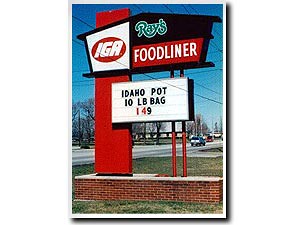This photograph captures an outdoor scene featuring a low red brick wall, situated on a patch of green grass. Atop this brick wall is a distinct sign display for Ray's IGA Food Liner. The main sign is designed to resemble a house, with a chimney-like structure on the left side. The left side of the sign is white with a red circle and the letters "IGA" in white, while the right side has a black background with the word "Ray's" in green and white, and "Food Liner" in a red rectangle with white letters beneath it.

Beneath this main house-shaped sign is a smaller, white rectangular billboard with customizable letters. It prominently advertises "Idaho P.O.T." in black letters, followed by "10 LB Bag" and the price "$1.49" displayed in red and black numbers. The background behind the signs features a blurry blue sky intersected by various power and telephone cables. Additionally, a road is visible with blurry cars, along with bare trees on the left side and more leafless trees further in the background.